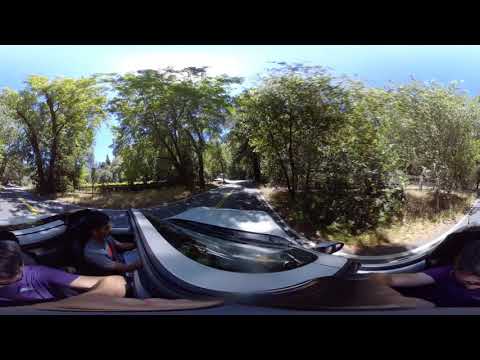The image depicts an outdoor scene, likely taken from inside a convertible or an open-topped vehicle, featuring three individuals driving along a paved road marked with a yellow stripe down the middle. The vehicle's perspective is slightly distorted, suggestive of a panoramic shot capturing a wider view. The sky is a bright, clear blue, indicating a sunny day. On either side of the road, tall, wispy green trees, casting heavy shadows onto the road, add to the lush, although not densely forested, surroundings. The area has ample vegetation, lending a somewhat park-like ambiance with patches of dirt visible beneath the trees.

In the foreground of the image, there is a curved structure extending from the center-left to the center-right, possibly part of the vehicle's dashboard. The three individuals in the vehicle appear to be fairly young, perhaps in their 30s. Two on the left are dressed in similar colored short-sleeved shirts, possibly purple, and seem to be looking downwards, engrossed in something in front of them. The driver, seated on the right and wearing a gray shirt, also faces this device, which might be a gadget or a screen integral to the vehicle's design. The detailed and vibrant environment highlighted by the clear weather and lush greenery creates a picturesque setting for this shared journey.